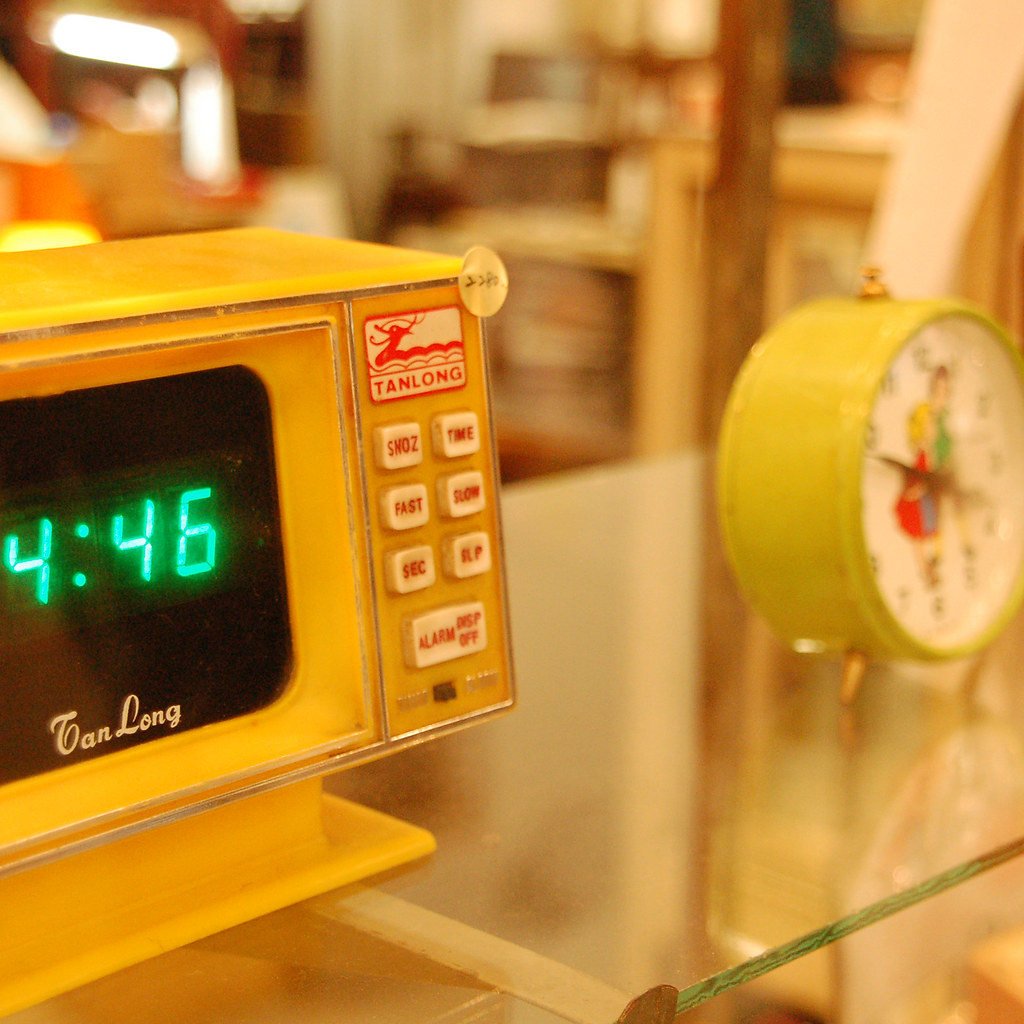This image features a modern digital alarm clock and a small vintage-style analog alarm clock, both placed on a sleek, translucent glass shelf. The main subject, the digital alarm clock, is housed in a glossy white, rectangular box supported by a matching boxy white stand with a wide, flat base. The clock face is black, displaying the current time "4:46" in bright blue digital numerals. The brand name, possibly "Ian Long," is printed on the upper part of the clock face in white letters, although the first letter of the name is highly stylized and somewhat unclear.

To the right of the digital readout is a panel of white buttons labeled in red with functions such as "SHOZ," "TIME," "FAST," "SLOW," "SEC," "BLP," "ALARM," and "BEEP OFF."

Adjacent to the digital clock is a small, round analog alarm clock with a striking yellow housing and a white face. The face of the analog clock features black numerals and multicolored figures, including illustrations of two women—one dressed in green and the other in red—though the image is slightly out of focus and part of the clock is out of frame.

The scene is set against a backdrop of a glass shelf, with various other objects in beige, cream, or wood tones faintly visible in the background.